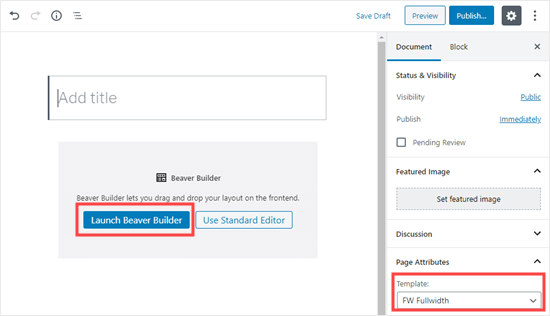This screenshot captures a user interface of a website builder tool where a user is configuring a draft for a new webpage. The interface displays several elements that facilitate the webpage creation process. 

At the top right corner, there are three primary action buttons: "Save Draft," "Preview," and "Publish." Adjacent to these, a gear icon button represents settings, and beside it, three vertical dots offer additional options. 

Directly below these buttons, the screen is segmented into two tabs: "Document" and "Block," with the "Document" tab currently active. 

Within the "Document" tab, various configuration options are detailed:
- **Status and visibility**
  - **Visibility:** Public
  - **Publish immediately**
  - **Pending review:** (a checkmark option that is not selected)
- **Featured Image**
  - **Set featured image:** (button)
- **Discussion**
- **Page Attributes**
- **Template**
  - **Selected template:** FW Full Width
  
On the left side of the interface, there is a preview pane showing what appears to be the draft of the website's layout. A placeholder field labeled "Add title" is visible and currently blank. Below this, there is an informational text about Beaver Builder which explains that it allows users to drag and drop layout elements on the front end. 

Two buttons are available for page editing: "Launch Beaver Builder" and "Use Standard Editor," with "Launch Beaver Builder" being highlighted by a red rectangle. Similarly, the “Template” button is also highlighted with a red rectangle, indicating areas of current focus or importance.

This detailed interface provides the user with comprehensive options and settings to meticulously draft and preview their website before publishing.